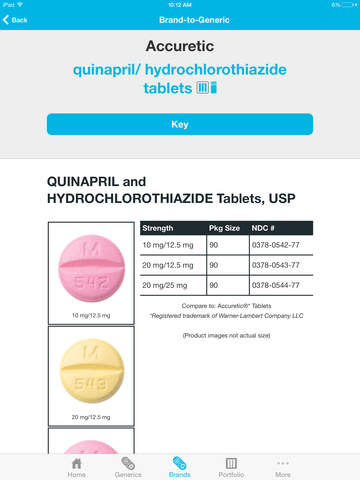Caption: 

"This image provides a detailed guide on selecting less expensive medication alternatives, specifically transitioning from brand-name to generic pills. The frame features a light blue stripe running from the upper left to the upper right. At the top center, the timestamp reads '12:12 a.m.' Below that, a back arrow accompanied by the label 'Brand to Generic' emphasizes cost-saving options by opting for generic medications over brand-name prescriptions.

Highlighted prominently, there is a large blue button with small letters inscribed with the symbol 'K,' possibly indicating a specific function or note. The prescribed pill in question is ACCURETIC, which consists of quinapril and hydrochlorothiazide tablets.

Further down, detailed information about the quinapril and hydrochlorothiazide tablets is displayed, indicating availability in dosages of 10 mg and 20 mg, typically packaged in quantities of 90 pills. On the left, images of the pills are shown: a pink pill marked with 'M over 542' and a yellow pill marked with 'M over 543.' The text urges users to compare these with ACCURETIC tablets for cost efficiency.

This visual aid highlights how the app assists users in selecting affordable medication alternatives, providing a practical and economical solution for accessing essential medication."